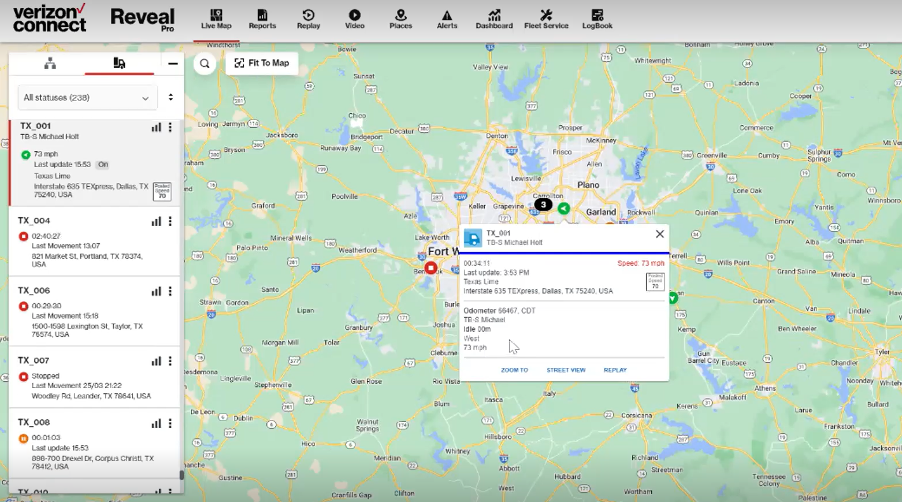The image showcases a detailed interface of the Verizon Connect application. At the top left corner, the Verizon Connect logo is prominently displayed in bold letters against a gray bar, accompanied by a comprehensive navigation bar to the right. This navigation bar includes labeled icons for various functionalities such as Reveal Pro, Live Map, Reports, Replay, Video, Places, Alerts, Dashboard, Fleet Service, and Log Book.

The main section of the image is dominated by a large map featuring regions shaded in green, with roadways marked in yellow, cities indicated in white, and bodies of water highlighted in blue. Centrally on the map, there is an overlay with the label "TX_001 TD-S Michael Holt," along with some additional, albeit blurry, information.

To the left of the map, there is a dropdown menu presenting a list of statuses. At the top of this menu is an icon depicting a computer connecting, followed by another indiscernible icon highlighted in red and underlined, signifying "Selected." Below this are several entries, each detailing different statuses. The first entry, "TX_001," is emphasized with a red line and selected. It indicates a speed of 73 MPH and an update timestamp of "1553." Subsequent entries, labeled "TX_004," "TX_006," "TX_007," and "TX_008," contain similar status information. Most of these entries are marked with a red stop sign, except for TX008 which is marked by an orange paw icon.